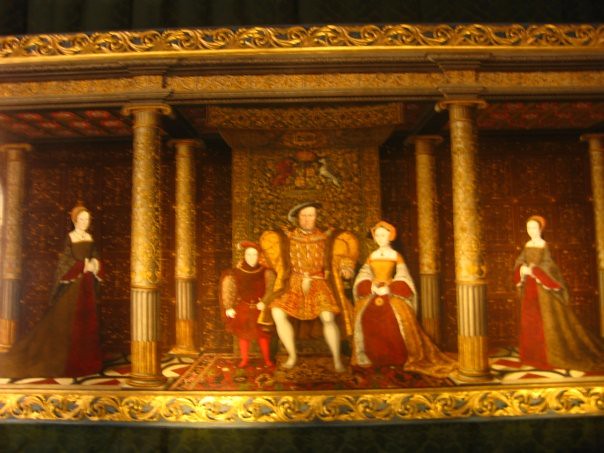In the photograph of a rectangular painting, the scene depicted is reminiscent of a Renaissance era, characterized by figures dressed in old-fashioned attire. The painting itself is surrounded by a black border, indicating that the entire artwork is not fully captured within the photograph. The setting appears to be an opulent room accentuated by gold columns and an intricately designed gold roof. Central to the composition is a figure, likely a king, possibly a King Charles or King Henry, who is the focal point of the scene. Surrounding this regal figure are various subjects, including a jester clad in red located towards the bottom left, and several ladies-in-waiting positioned to his right and left. The painting's floor features ornate circular tiles in a striking palette of black, red, and white, with the king's area highlighted by a large Persian-style rug. Rich hues of gold, red, and yellow dominate the color scheme, adding to the painting's luxurious and historical ambiance.